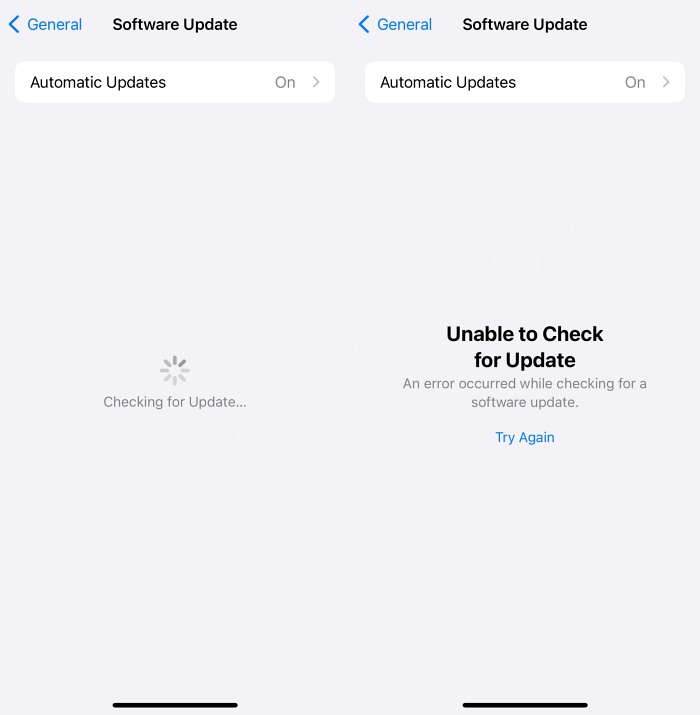The image consists of two adjacent smartphone screenshots set against a light gray background. The left screenshot displays the software update settings interface. At the top of the screen, in a blue font, it reads "General" with a left-pointing arrow. Directly next to it, in black text, it says "Software Update." Below this heading is a white rectangular box that contains the text "Automatic Updates" on the left and "On" in a gray font on the right, alongside a right-pointing arrow. In the center of the screenshot, a spinning gray wheel is visible with the text "Checking for update" underneath it.

The right screenshot mirrors the layout of the left one at the top, showing "General" in blue with a left-pointing arrow and "Software Update" in black text. However, this screenshot shows a different status in the white box. While "Automatic Updates" is still indicated as "On," the middle section contains bold black text stating, "Unable to Check for Update." Below this, smaller gray text reads, "An error occurred while checking for a software update." At the bottom, a blue prompt says "Try Again."